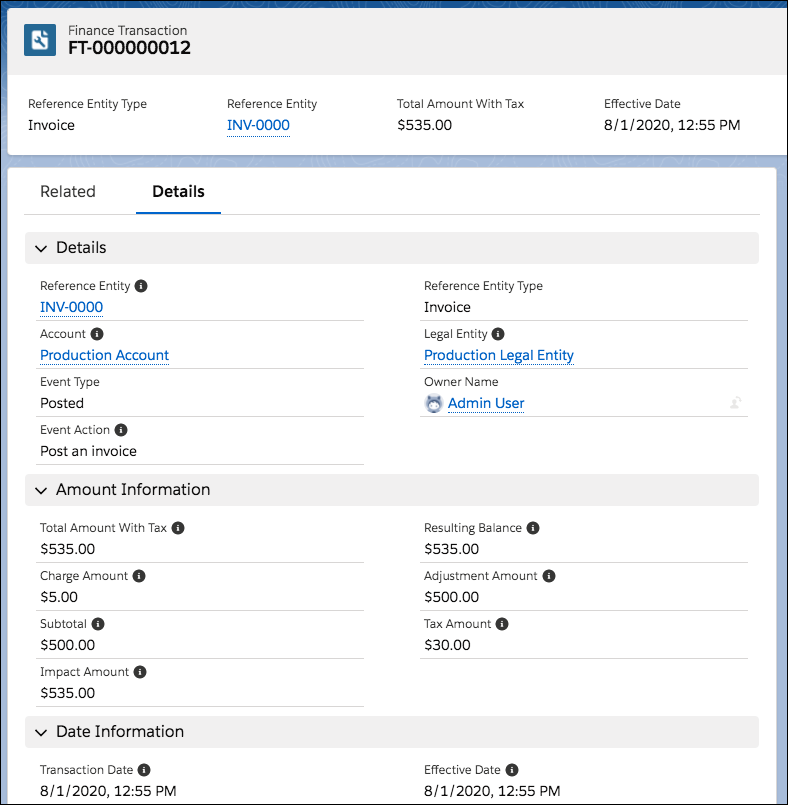Screenshot Description for a Finance Transaction Page:

The image is a screenshot of a finance transaction details page. At the top, there is a grey bar containing a blue logo. The logo depicts a white piece of paper with a wrench inside it. Next to the logo, the title "Finance Transaction" and the serial number "FT-0000000012" are displayed.

Below the header, the page lists various details about the transaction. The following information is provided:

- **Reference Entity Type**: Invoice
- **Reference Entity**: INB-0000
- **Total Amount with Tax**: $535
- **Effective Date**: August 1st, 2020, at 12:55 PM

The page presents two options: "Search for Related" and "Details." The "Details" option is highlighted in black, indicating the user is currently viewing this section. 

In the "Details" section, which is under a grey bar with a downward arrow, multiple attributes related to the transaction are listed, including:
- Reference Entity Account
- Event Type
- Event Action
- Reference Entity Type
- Legal Entity
- Owner Name

Another grey bar titled "Account Information" follows, providing a breakdown of financial figures:
- Total Amount with Tax
- Charge Amount
- Subtotal
- Impact Total
- Resulting Balance
- Adjustment Amount
- Tax Amount

At the bottom, a grey bar titled "Date Information" with a downward-pointing arrow details further timelines related to the transaction:
- Transaction Date
- Effective Date

Each section is clearly delineated by grey bars, ensuring the details are neatly organized and easy to navigate.